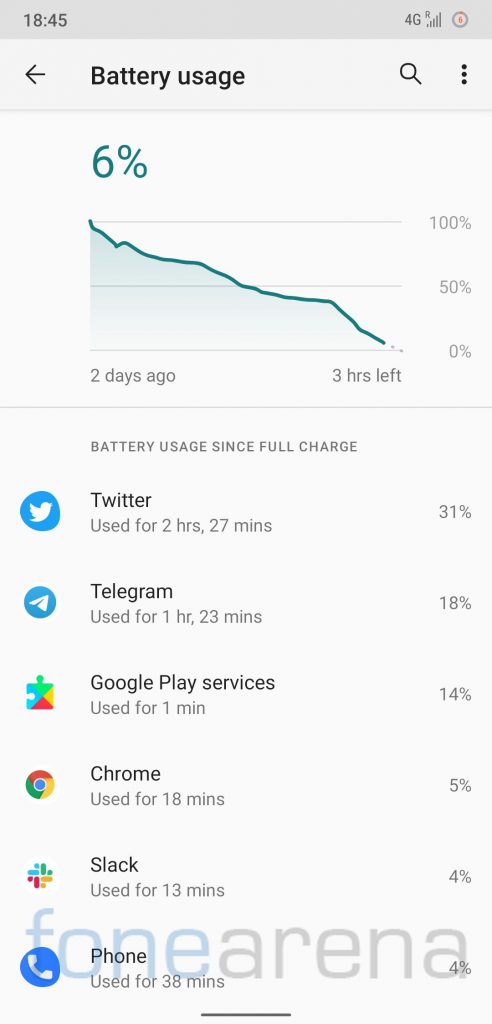The image displays a smartphone screen open to the Battery Usage section. Dominating the top portion is a dark teal line graph detailing the battery percentage over time. Beginning at 100% two days ago, the graph illustrates a steady decline to 6%. Approximately a day ago, the battery level was around 50%, continuously decreasing to the current state. The graph indicates an estimated 3 hours of battery life remaining.

Below the graph, the section labeled "Battery usage since full charge" itemizes the app usage statistics:
- **Twitter:** Used for 2 hours and 27 minutes, consuming 31% of the battery.
- **Telegram:** Used for 1 hour and 23 minutes, contributing to 18% of battery drain.
- **Google Play services:** Active for 1 minute, using 14% of the battery.
- **Chrome:** 18 minutes of usage accounting for 5% of the battery.
- **Slack:** 13 minutes of activity, resulting in 4% battery usage.
- **Phone:** Utilized for 38 minutes, comprising 4% of the battery consumption.

At the bottom of the image, the text "Phone Arena" is visible, suggesting the source or branding associated with the content.